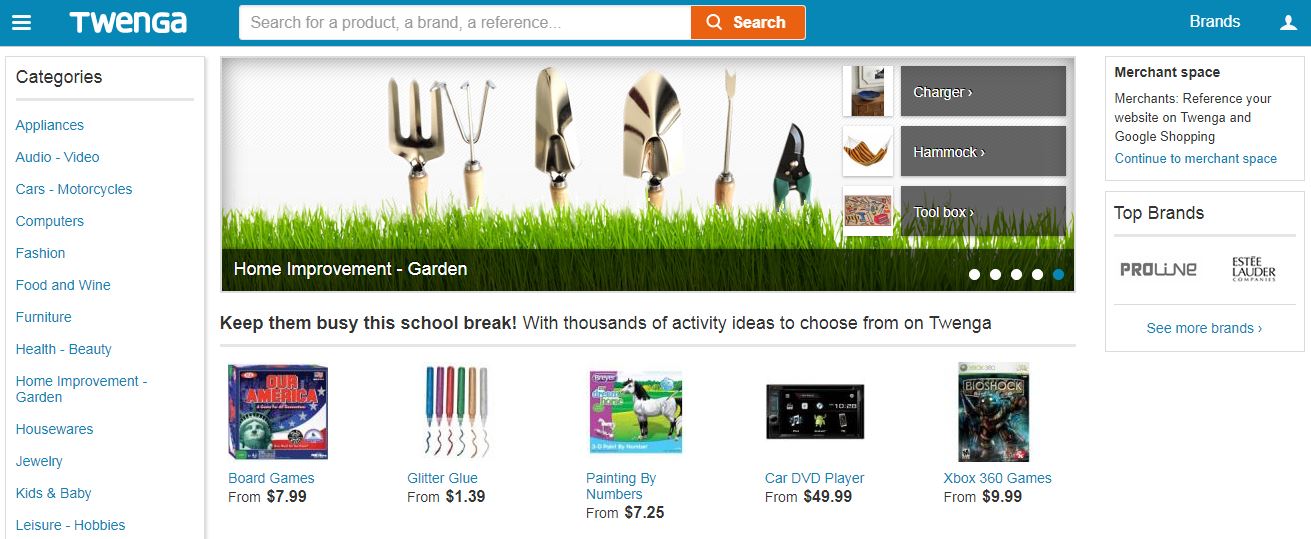This web page is from the shopping website TWENGA. The site features a header with "TWENGA" prominently displayed in white letters against a blue banner at the top of the page. Centrally located on this blue banner is a search box with a white background and an adjacent blue search button.

Beneath the header, the site showcases an image of small handheld garden tools, laying on a patch of green grass, suggesting a focus on gardening items at the moment. 

The main content of the page lists various products available for purchase. Items displayed include board games starting at $7.99, glitter glue for $1.39, painting by numbers kits from $7.25, car DVD players starting at $4.99, and Xbox 360 games from $9.99. This diverse selection indicates that TWENGA offers a wide range of products, from garden tools to video games, craft supplies, and automotive accessories.